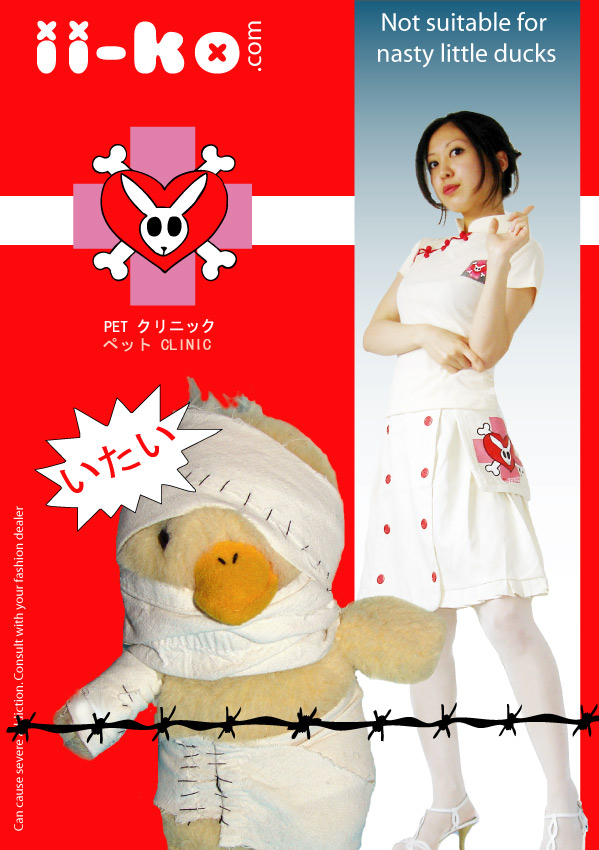The image appears to be a promotional advertisement for a Japanese nurse cosplay outfit by the company II-KO. The label features a distinctive aesthetic with a color scheme predominantly of red and white. The II-KO logo is composed of stylized elements, including a pink nurse's cross behind a red heart with a caricature of a white rabbit head, black hollow eyes, and crossbones. This emblem is also present on the breast and side pockets of the costume.

The costume itself includes a white, short-sleeved top with a popped collar, a skirt that reaches just above the knees adorned with a panel of four buttons on each side, white stockings, and midsize white heels. The model is a young woman of East Asian descent with medium-toned skin and black hair styled short, lending an authentic touch to the Japanese nurse theme.

Additional elements in the advertisement include an injured stuffed toy duck, wrapped in bandages covering its eye, arm, and lower body, symbolizing the medical theme. The duck appears against a backdrop that transitions from an orange background on the left to a bluish-white background on the right, bordered with orange. Above the company's name "KO," there's a playful motif featuring two white X's, vertically oriented slashes, and a hyphen. The topmost 'O' in "KO" contains a red X, with ".com" extending vertically from it.

Beneath the logo, there is purple "X" mark with crossbones running through it, combined with a rabbit head. There's also white text underneath this emblem that is not clearly legible. The tagline "not suitable for nasty little ducks" is prominently displayed within a white bubble with red writing and triangular edges. Black barbed wire imagery runs horizontally across the chest area of the stuffed duck within the advertisement, adding an edgy contrast to the overall design.

Altogether, the intricate details and thematic elements create a vivid and appealing promotional ad that aligns with Halloween or cosplay markets.